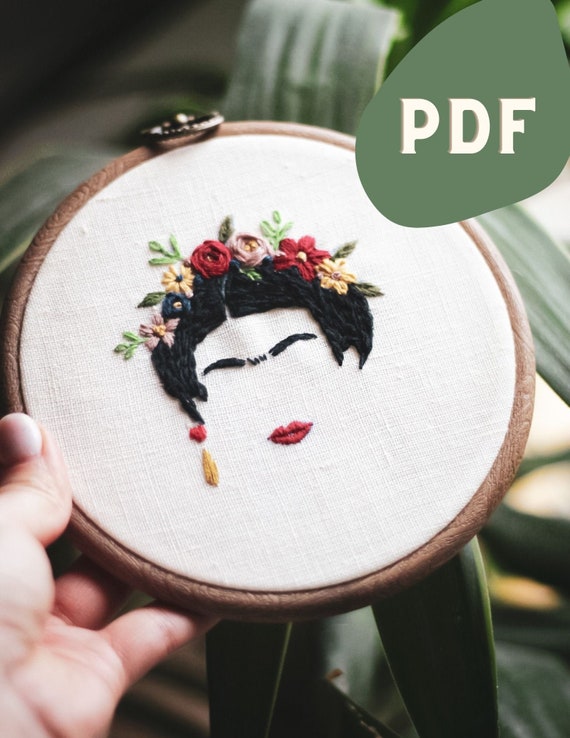This detailed color photograph showcases a hand emerging from the bottom left, holding a round brown wooden embroidery hoop with a brass-colored hook at the top. The hoop frames a cream-colored fabric adorned with an intricate embroidery of Frida Kahlo's iconic features: stark black hair parted in the middle, dark black interconnected eyebrows forming almost a unibrow, and vivid red lips. Her hair is festooned with a crown of multicolored flowers, including red, yellow, pink, and blue blooms among green leaves. The backdrop, rendered in soft green tones, appears out of focus. In the upper right corner, a green, amoeba-shaped block features the cream-colored text "PDF". A plant is faintly visible in the background, adding to the image's natural aesthetic.